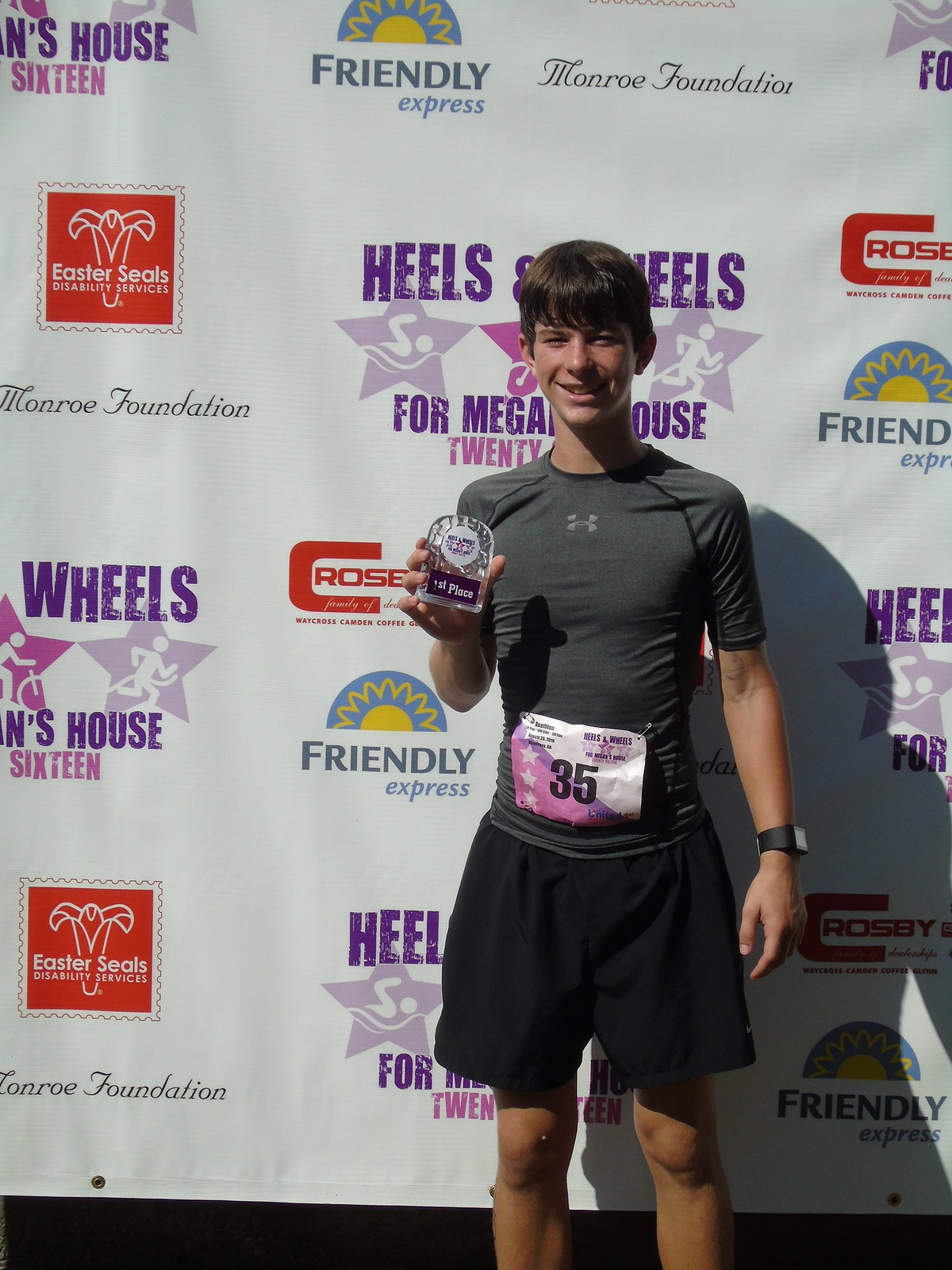In the image, a young boy, likely in his early teens, stands smiling at the camera at a sports event. He has brown hair and is dressed in a tight-fitting gray athletic t-shirt with the number 35 pinned to the front, along with black shorts. A wristwatch adorns his left wrist. He proudly holds a small silver plaque that has a purple banner at the bottom indicating "first place." 

The background features a full-length banner filled with various advertisements. Notable sponsors include Easter Seals, displayed prominently in a red box with white lettering and an icon, as well as the Monroe Foundation in cursive below it. Friendly Express appears multiple times across the banner. Additional details include logos likely representing "Heels For Wheels for Megan's House" and other sponsors. The young boy's euphoric expression and his first-place award highlight his achievement, set against a backdrop of sponsor logos and vibrant advertisements.